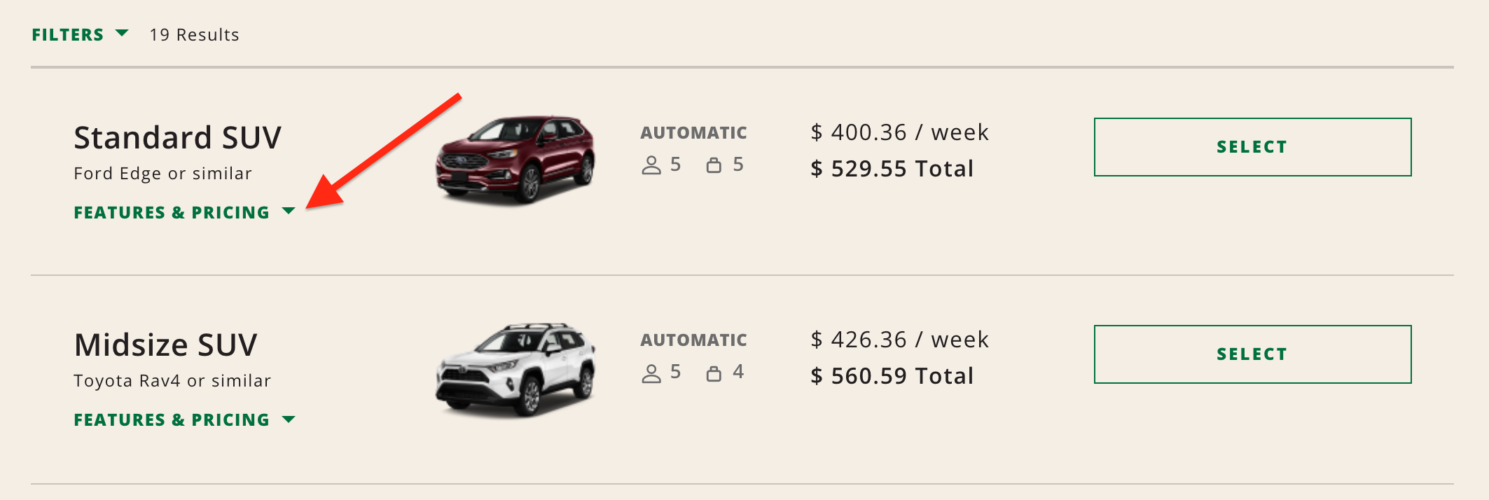This screenshot illustrates search results on a website displaying available SUVs. The background is a light beige at the top left corner. A drop-down menu labeled "Filters" indicates there are 19 results. Below this is a horizontal black line.

The first entry is labeled "Standard SUV Ford Edge or Similar" and features a drop-down menu for "Features and Pricing." A red arrow, photoshopped into the image, points to the drop-down menu. Next to the arrow is a photo of a black SUV. The detailed information beside the photo indicates "Automatic," "Seats: 5 People," and includes an icon of a shopping bag labeled "5" (the meaning of this icon is unclear). The cost details are "$400.36 per week" and "$529.55 total." A "Select" button is placed adjacent to these details.

The second entry is for a "Midsize SUV Toyota RAV4 or Similar" and also includes a drop-down menu for "Features and Pricing." Beside this is a picture of a gray Toyota RAV4. The vehicle details list "Automatic," "Seats: 5," and again a shopping bag icon labeled "4." The pricing information states "$426.36 per week" and "$560.59 total." A "Select" button is available next to these details.